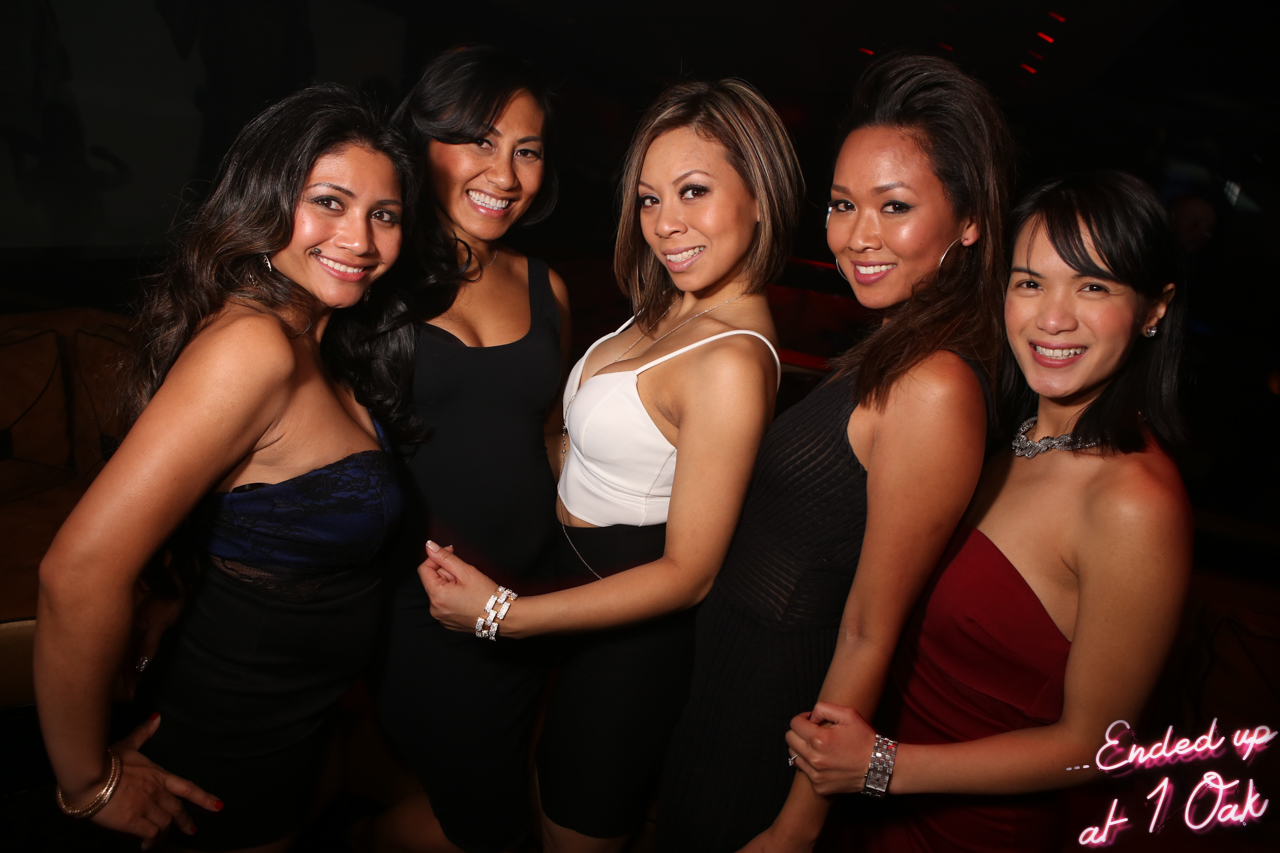This photographic image, likely taken indoors at a venue called One Oak as indicated by the cursive white text in the bottom right corner, captures five women dressed for an upscale evening out. The women, who appear to be of diverse ethnic backgrounds—including Asian, African-American, and possibly Hispanic or Middle Eastern—are elegantly posed and smiling, exuding a sense of fun and camaraderie. From left to right: the first woman wears a black, sleeveless or strapless dress and looks toward the camera; next to her, another woman also in a black dress faces the camera. The center woman, standing out in a white spaghetti strap tank top showing cleavage, pairs it with a black skirt. The fourth woman dons a minimalistic black dress, while the fifth woman on the far right wears a striking red tube top, adorned with a bracelet, wristwatch, ring, and a green jean necklace. All are in their early to mid-30s with darker hair and complexions, ready for a lively night at the club.